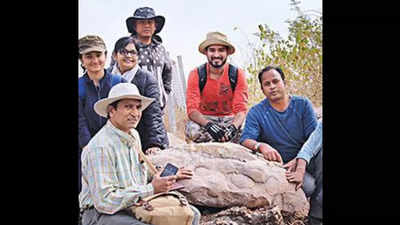The image is a small, low-quality, horizontally rectangular, full-color photograph taken outdoors during the daytime using natural light. The colors in the image have significantly faded. The photograph is nestled within a black border that runs vertically along the left and right sides. 

The central focus is on a square photograph depicting a group of seven people gathered around a large, light brown rock that they appear to be posing with, possibly indicating it as an archaeological find or significant natural formation. The backdrop features a clear blue sky, and a green bush is visible in the upper right-hand corner, while the bottom foreground displays the prominent rock.

Out of the seven individuals, whose faces are brightly smiling, four are men and two are women with the hand of a seventh person just visible. The group consists of individuals in varying postures: some are sitting, some are standing, and one man is kneeling in front of the rock on the left-hand side, holding a phone in his hand. He’s dressed in gray pants and a light blue and red pastel plaid long-sleeve shirt with a round white hat. To his left, two women wearing long dark navy blue jackets can be seen, one with an olive green hat. 

On the right-hand side, there are two men; one is wearing a long sleeve blue shirt, the other a long sleeve red shirt paired with a hay-colored round hat. Behind the group, another man, identifiable by his jacket and hat adorned with white stars, sits observing the scene. The entire group exudes a joyous camaraderie, epitomizing a moment of exploration and shared excitement.